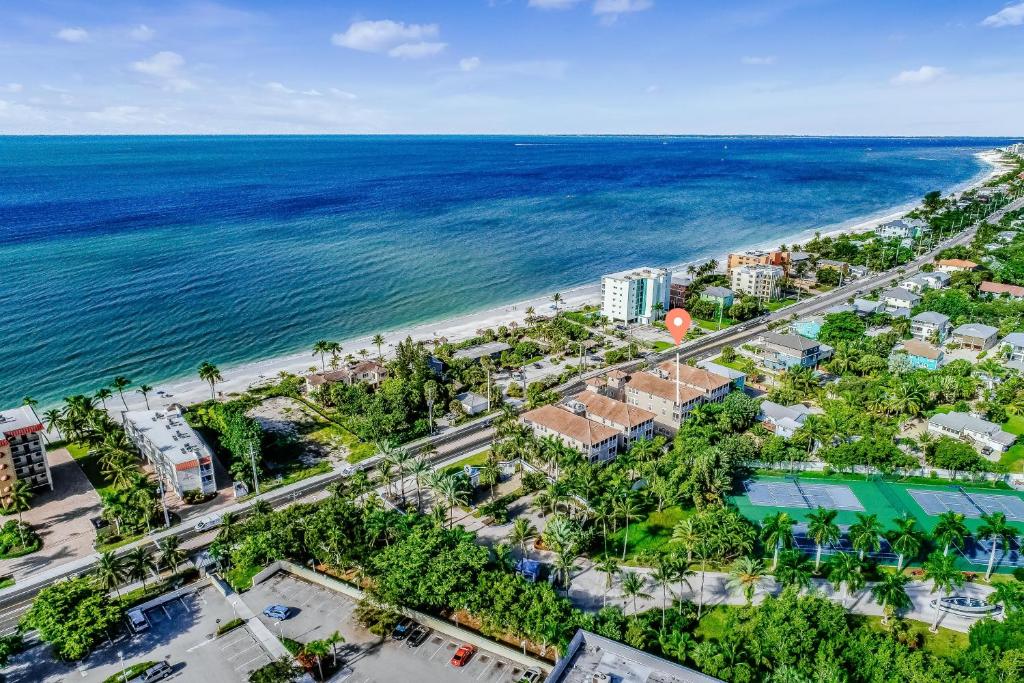This is a detailed color aerial photograph of a stunning beachfront area, likely a resort situated on an island or in a coastal region such as California. The image captures a broad stretch of vibrant blue ocean, reflecting various hues from deep blue to turquoise, indicative of sunlight and possibly a coral reef beneath the surface. The sky is a light blue adorned with fluffy white clouds, contributing to the serene ambiance. 

The beach itself is a white sandy expanse running diagonally from the bottom left to the upper right corner, flanked by a series of hotels, bungalows, and homes. A distinguishable orange pin with a white circle points to a specific property almost at the center of the image, suggesting it could be a prominent condo or rental property. 

In the landscape behind the beach, rich green vegetation intersperses with buildings, providing a lush backdrop. A road separates the beachfront structures from another cluster of homes and condominiums further back. The lower right corner of the image features a tennis court, while a parking lot is visible in the lower left. Additionally, elements suggesting a golfing range are present among the various buildings, adding to the resort-like atmosphere. Cars are discernible on the roads, adding a hint of bustling activity to the tranquil setting. The horizon line is near the top of the image, emphasizing the far-reaching view of this picturesque locale.